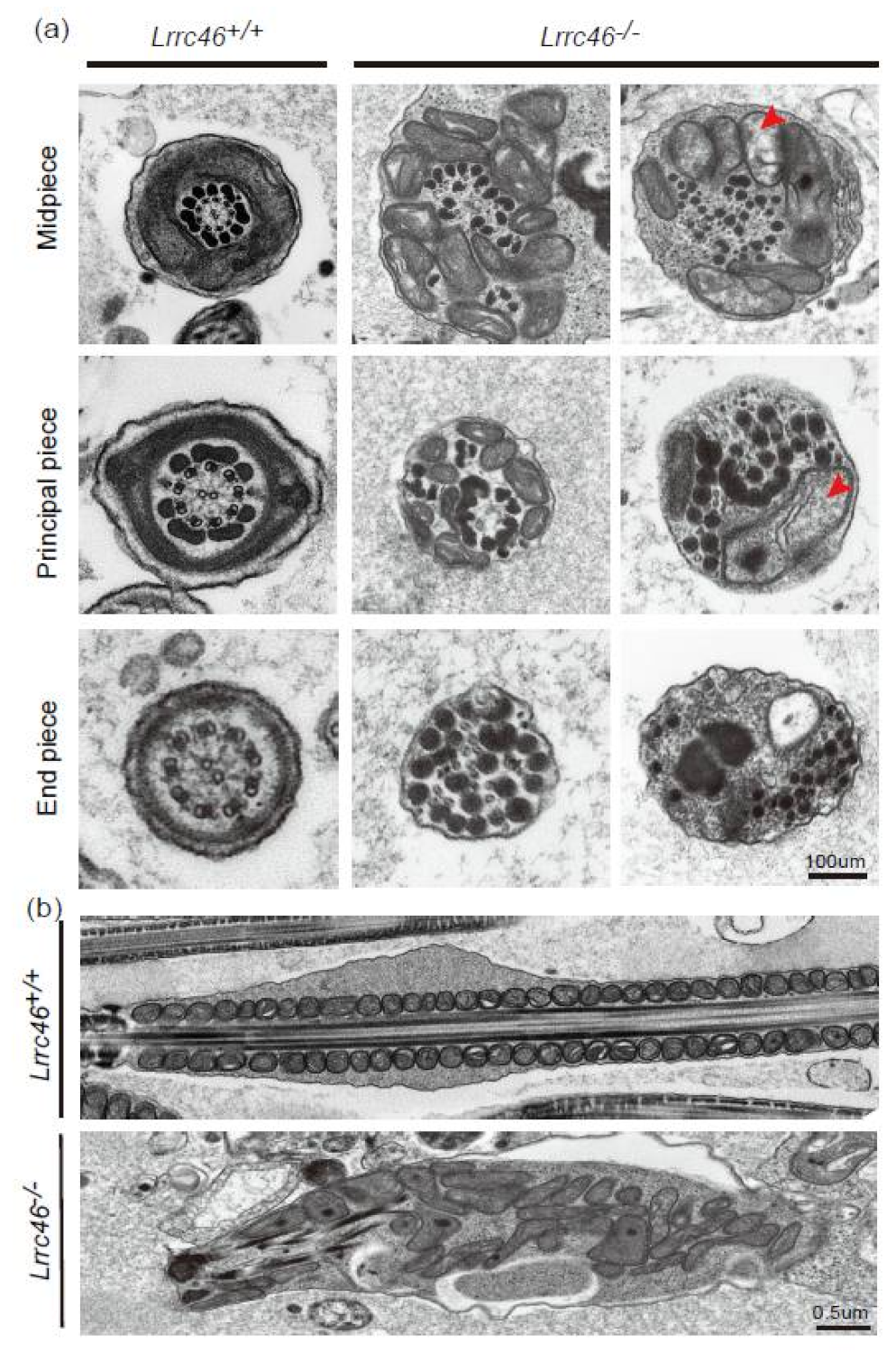This vertical black-and-white image presents a detailed series of what appear to be highly magnified, possibly microscopic images or meticulous drawings of fossilized structures. The composition features eleven distinct sections. At the top, there are nine square images arranged in a grid, each labeled on the left side with terms such as "mid-piece," "principal piece," and "end piece," suggesting these are various cross-sections or phases of the specimen under study. Below this grid, there's a rectangular picture that intriguingly resembles a stone fossil or a zipper-like stone artifact that appears sheared in half. At the very bottom of the image, there's a depiction of what looks like either a fossil embedded in a rock or an intricate rock design. Some annotations include unexplained letters and numbers. Notably, while the primary palette is black and white, there are subtle touches of red, potentially to highlight specific details or sections.